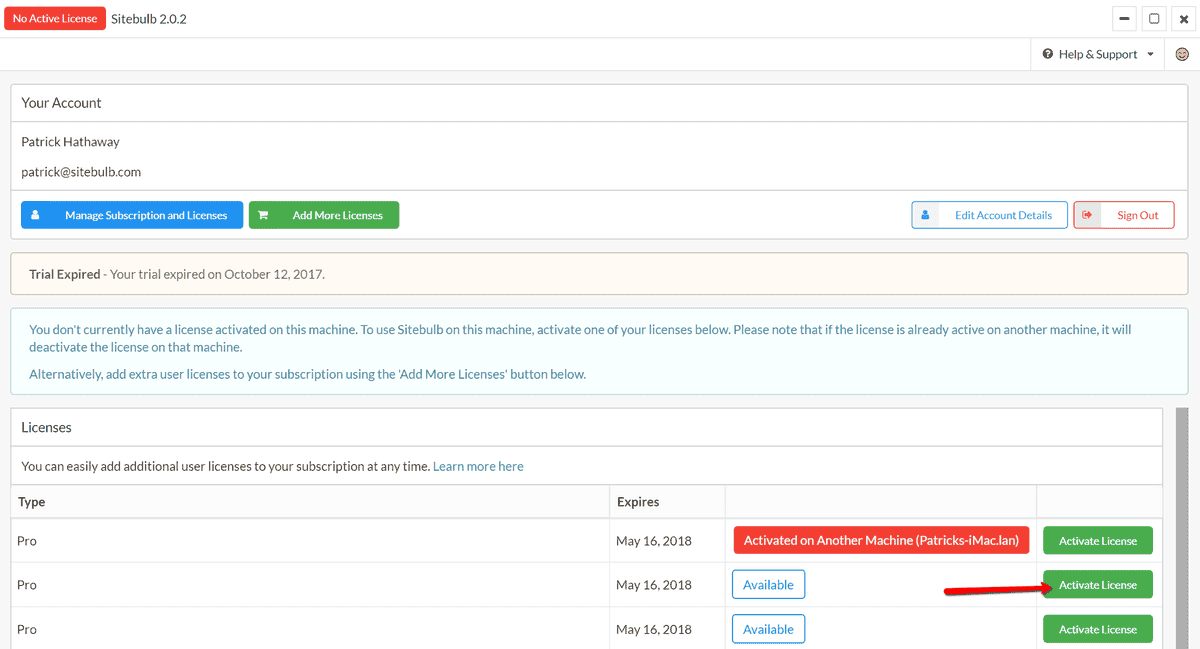On the web page, the user interface is organized efficiently with various sections clearly designed for account management and license control. 

- **Top Left Corner**: There is an orange box with white text that reads "No Active License". In front of this box, black text displays "SiteBulb 2.0.2" (the version number may be slightly unclear due to small text size).

- **Top Right Corner**: There are three icons for window management:
  - Minimize icon
  - Full-screen icon
  - Close (X) icon

- **Below the Header**: A white bar spans across the page. On the far right of this bar, there is a white tab featuring:
  - A gray circle with a white question mark, labeled "Help & Support" with an arrow indicating more options.
  - A yellow smiling emoji face icon next to it.

- **Account Information Section**: 
  - A white background area displaying "Your Account" with the following details:
    - Name: Patrick Hathaway
    - Email: patrick@sitebulb.com
  - Below the account name and email, there are two buttons:
    - A blue button on the left with a silhouette icon labeled “Manage Subscription and Licenses”
    - A green button with a card icon labeled “Add More Licenses”

- **Right Side Buttons**: 
  - Next to the account information, there are two buttons:
    - A button with a blue outline and text that says "Edit Account Details"
    - A button with an orange outline and text that says "Sign Out"

- **Trial Information Section**: 
  - A tannish colored bar that reads "Trial Expired: Your trial expired on October 12, 2017"
  - Below this, a blue box states: "You don't currently have a license activated on this machine. To use SiteBulb on this machine, activate one of your licenses below. Note that if the license is already active on another machine, it will deactivate the license on that machine. Alternatively, add extra user licenses to your subscription using the ‘Add More Licenses’ button below."

- **Licenses Section**: 
  - A white bar with the heading "Licenses" followed by a note in blue text: "You can easily add additional user licenses to your subscription at any time. Learn more here."
  - A table below this section:
    - The header row is gray, with columns labeled "Label Type" and "Expires"
    - First row: 
      - “Type: Pro” and “Expires: May 16, 2018” 
      - An orange tab with white text stating "Activated on another machine - Patrick's iMac"
      - A green "Activate License" button
    - Second row:
      - “Type: Pro” and “Expires: May 16, 2018”
      - A white box with a blue trim labeled "Available"
      - A red arrow pointing at the green "Activate License" button
    - Third row:
      - “Type: Pro” and “Expires: May 16, 2018”
      - Similar to the second row, featuring an "Available" button and a green "Activate License" button

This detailed layout provides a comprehensive view of the user’s account and license management interface on the SiteBulb web page.